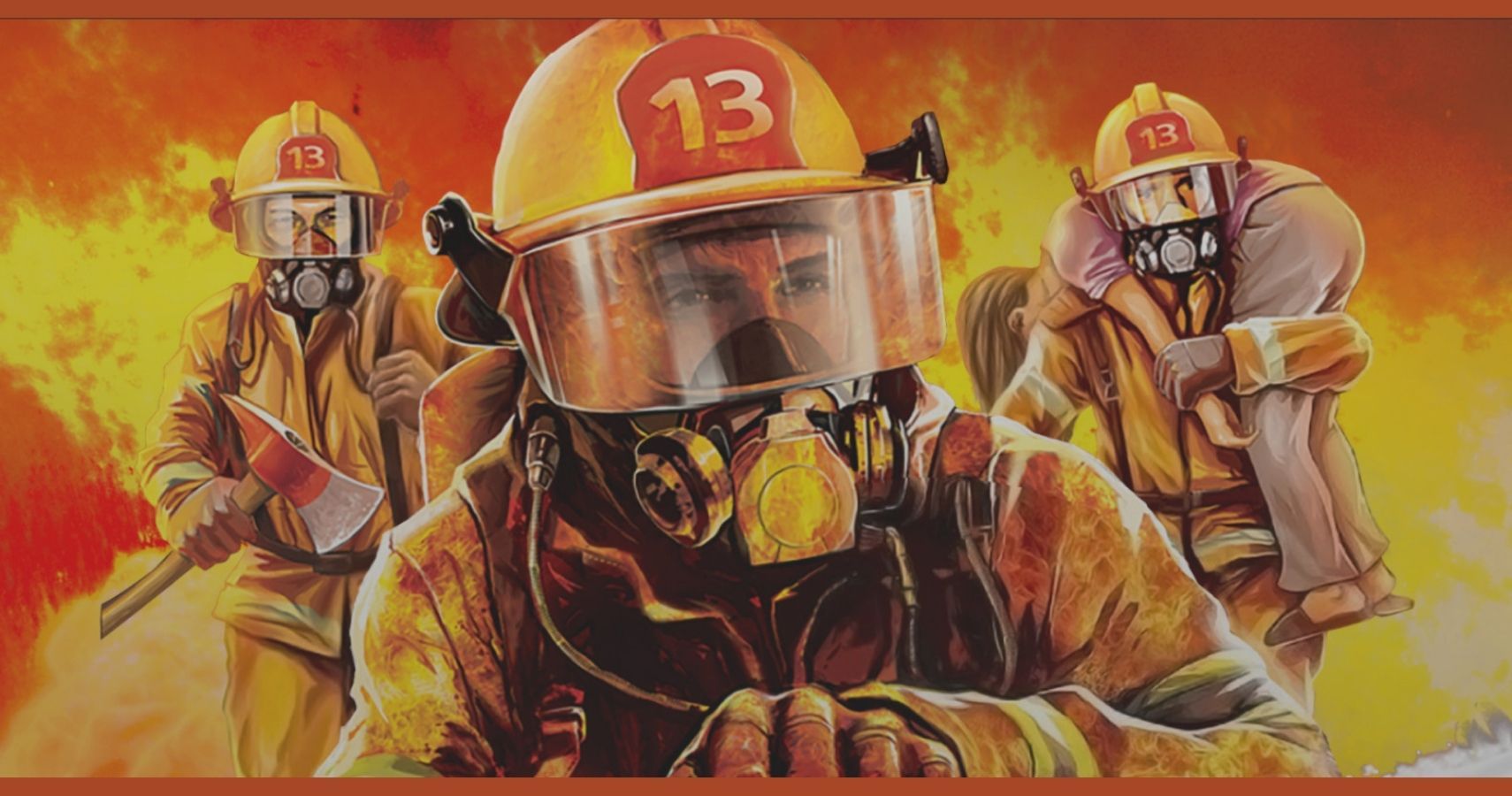In this vibrant, detailed illustration, three firefighters, adorned in their full firefighting gear including yellow jackets, yellow pants, and helmets marked with the number 13, are depicted heroically running from a roaring inferno blazing behind them. The firefighter on the right side is seen with a girl slung over his shoulder; she appears to be wearing pajamas and slippers, with her hair draped over his shoulders, obscuring her face. The firefighter on the left brandishes a machete, while all three wear breathing masks and visors to shield themselves from the intense heat and smoke. The chaotic scene is filled with flying embers and a wall of flames, emphasizing the dangerous and wild nature of the fire they are escaping. The firefighters are forward-focused, portraying an image of determined bravery and urgency as they rescue the girl from the perilous blaze.